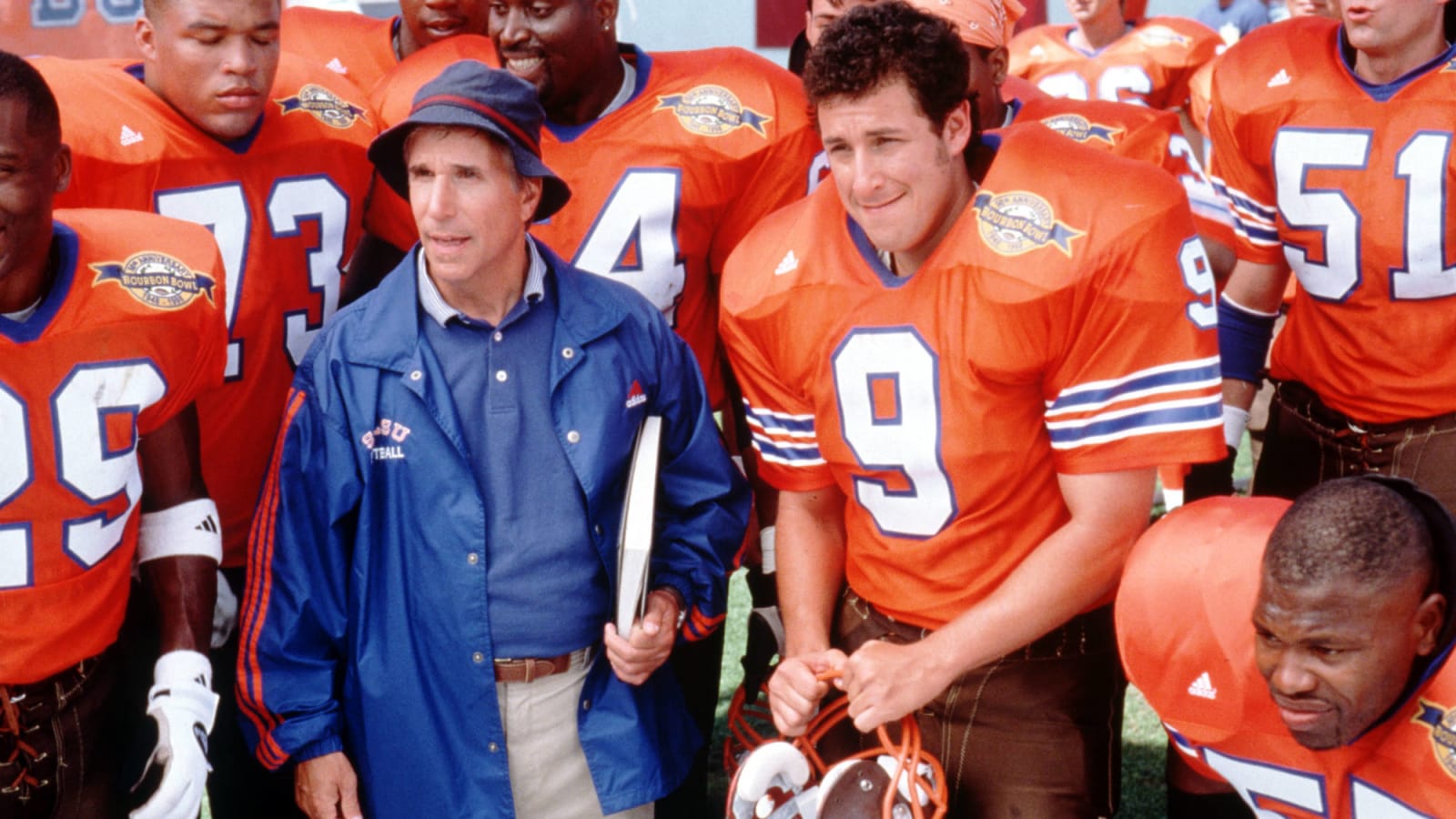This detailed screenshot from the movie "The Waterboy" features a group of football players and their coach in mid-action. Front and center is Adam Sandler in an orange jersey with blue and white stripes, prominently displaying the number 9. He is holding his orange helmet, which matches his uniform. Beside him stands Henry Winkler, playing the coach, outfitted in light tan khaki pants, a brown belt, a navy blue polo shirt, and a blue windbreaker jacket with red stripes. Winkler also sports a blue bucket hat with a red stripe and has a clipboard tucked under his left arm. Encompassing them, approximately seven to eight other players are clad in matching orange jerseys with retro brown pants, and one player to the left is distinctively wearing white gloves and a white Adidas armband. Visible jersey numbers include 29, 73, 4, 9, and 51. The scene captures a moment of anticipation, with Adam Sandler's expression reflecting a mix of focus and subtle tension.